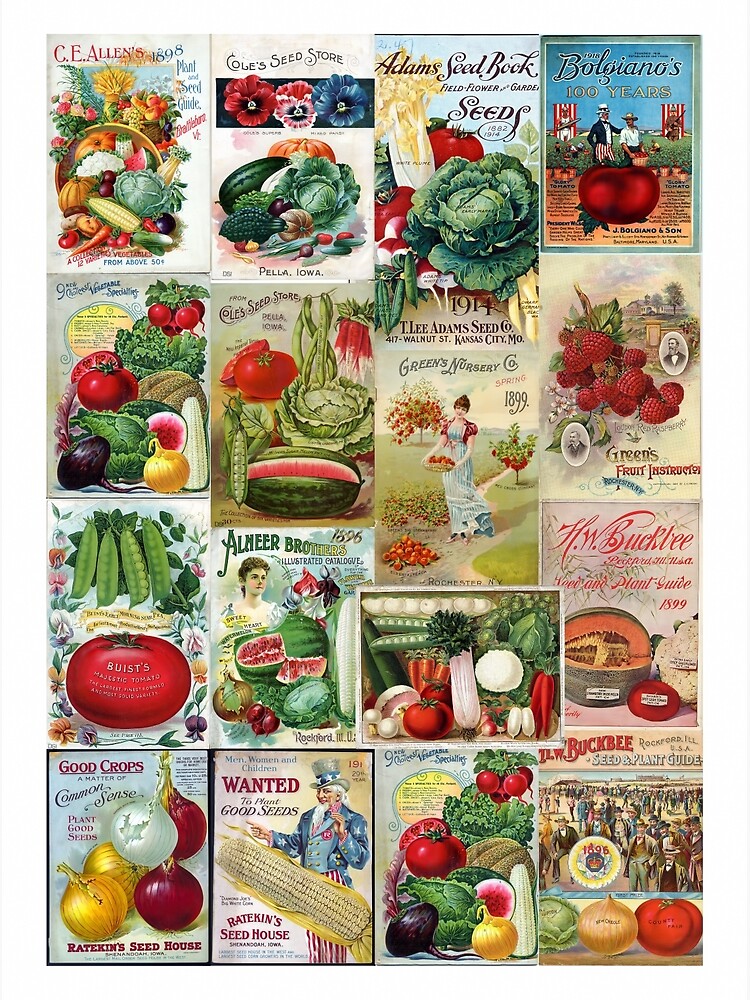This detailed collage depicts a vibrant collection of 16 vintage seed catalog posters, meticulously illustrating various fruits, vegetables, and flowers from different seed companies. The imagery draws the viewer's attention with an array of colors – from the lush greens of cabbages and lettuces to the deep reds of tomatoes and strawberries, the golden yellows of corn and onions, and even the subtle hues of cauliflowers and watermelons.

Each poster, arranged in a 4x4 grid, boasts unique and period-specific artwork, filled with rich, vibrant tones as well as some muted tans. Names like "C.E. Allen's 1898," "Cole's Seed Store," "Adam's Seed Book," "Green's Nursery Spring 1899," and "Raitkin's Seed House" are prominently featured, alongside slogans and detailed illustrations representative of late 19th to early 20th-century advertising.

The prints range from depictions of individual vegetables like cucumbers, raspberries, cantaloupes, and pumpkins to more elaborate scenes, such as a young woman gathering fruit in an orchard and an iconic Uncle Sam holding an inviting cob of corn with a call to action: "Men, Women, and Children WANTED to Plant Good Seeds – Raitkin's Seed House." The backdrop is an engaging assortment of colors, including blues, whites, greens, and yellows, enhancing the nostalgic appeal.

This collage not only showcases the horticultural variety but also reflects the diverse marketing styles of a bygone era, making it a rich, visual tapestry of agricultural heritage.